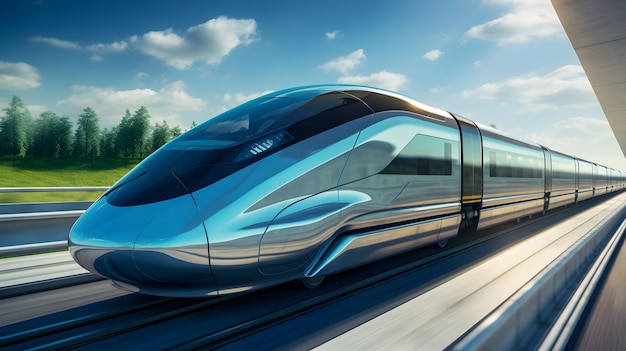The image features a sleek, modern high-speed train designed with a bullet-like shape to enhance aerodynamics. The train's body is a gleaming silver with a striking black front mask and black-tinted glass windows that run along its sides. It glides on a shiny silver-gray railroad track. The background showcases a serene blue sky adorned with thick, fluffy white clouds resembling cotton balls. Below the horizon, vibrant light green grass stretches out, accompanied by tall trees brimming with lush green leaves, adding to the picturesque scenery.